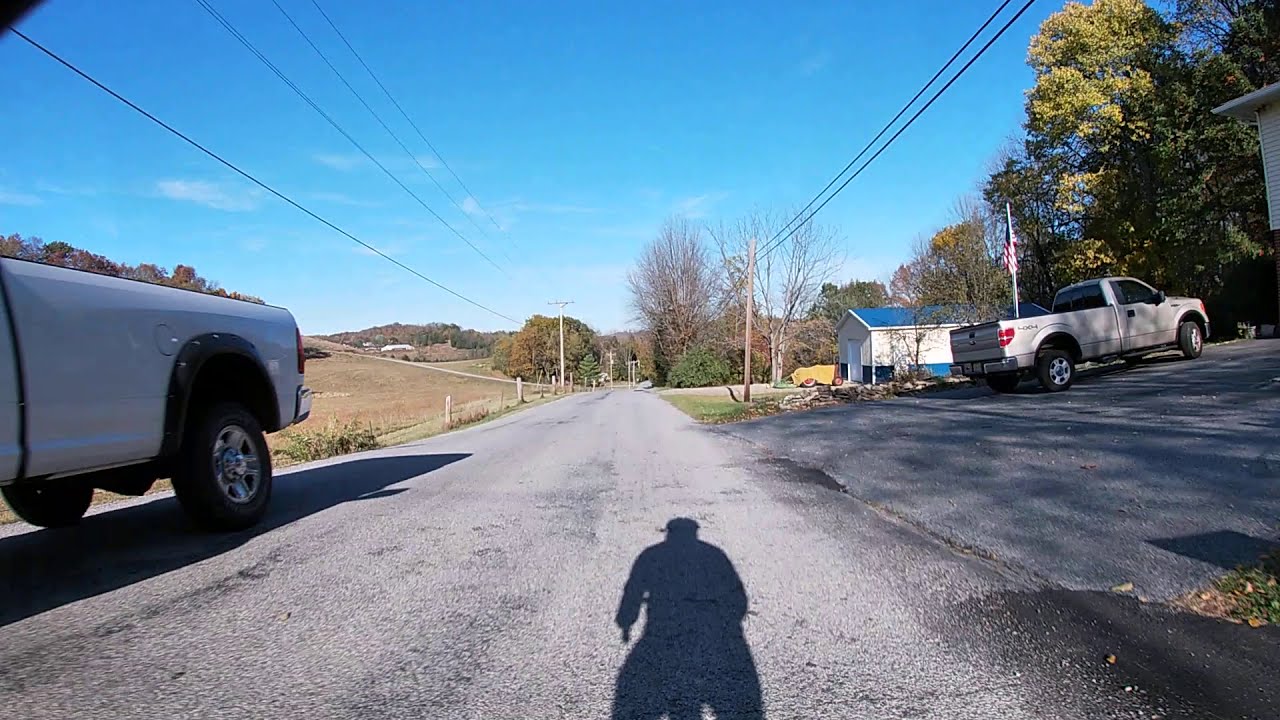The image captures a picturesque, sunny day on a narrow country road lined with telephone poles and surrounded by early autumn scenery. The central feature is the prominent shadow of a man, seemingly riding a bicycle or motorcycle, cast onto the asphalt road. On the left side of the road, a white pickup truck is parked, while on the right side, another white pickup truck rests in a driveway that leads to a white house adorned with a blue roof. An American flag flutters on a flagpole next to the house. The landscape in the background reveals rolling, slightly hilly terrain dotted with numerous trees, some of which are beginning to turn yellow, indicating the transition from summer to fall. The sky is a clear, vibrant blue with only a few wispy clouds, adding to the serene and tranquil rural atmosphere conveyed by the image.